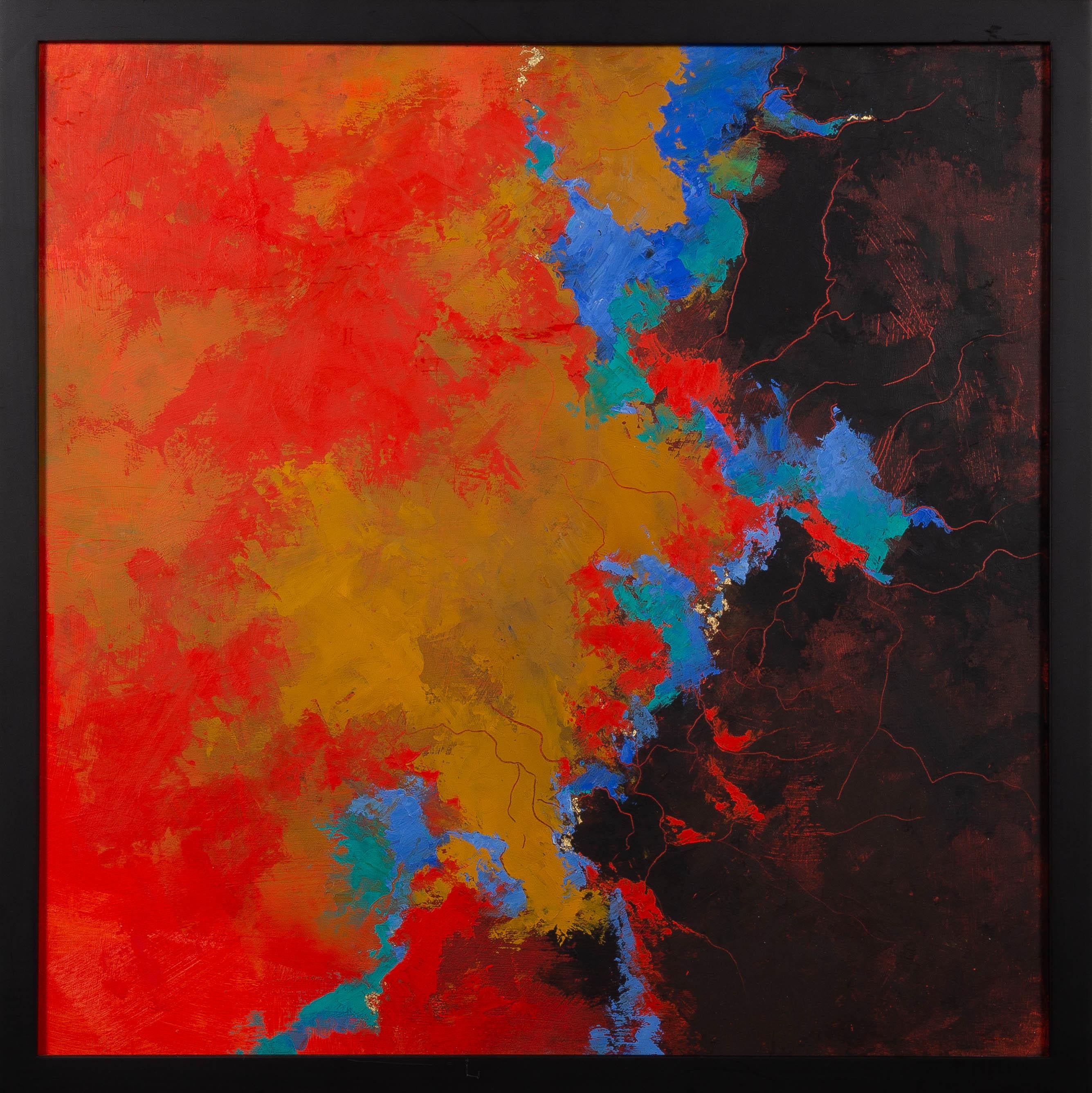The image is a digital screenshot of a framed piece of art, primarily dominated by a black wooden frame. The artwork within features a striking combination of colors. The left portion of the painting is mainly red and yellow, or orange and red, giving it a vibrant appearance. The right side is predominantly black with intricate vein-like patterns of red, adding a dramatic contrast. A blue and green area runs vertically through the center, resembling a river that separates the two halves. This central strip provides a harmonious balance to the composition. The overall blend of colors includes black, red, blue, green, and touches of yellow and orange, creating a multifaceted and dynamic visual experience.